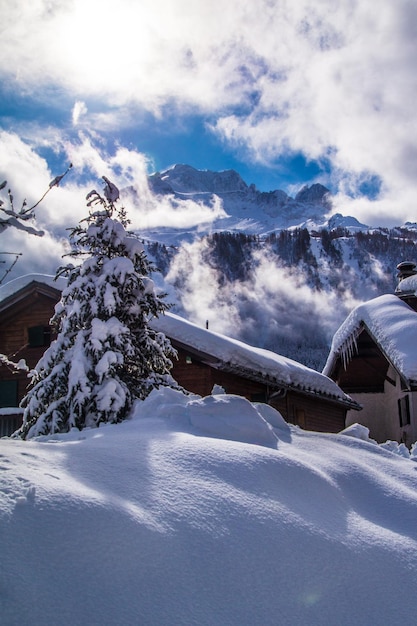The photograph showcases a picturesque winter landscape, dominated by towering, jagged mountain peaks in the background, possibly characteristic of the Rocky Mountains or a Swiss Chalet setting. The majestic mountains are capped with varying textures of fluffy white clouds. In the foreground, there stands a grand, snow-laden tree resembling a Christmas tree, under which two distinct houses are nestled. One house is brown, and the other is white or beige, both topped with thick layers of snow and adorned with icicles hanging from the roofs' edges. Between the houses and the mountains, stretches a dense forest of spruce or pine trees, all blanketed in pristine snow. The entire scene is enveloped in deep snow mounds, completing this idyllic, remote winter resort-like atmosphere.